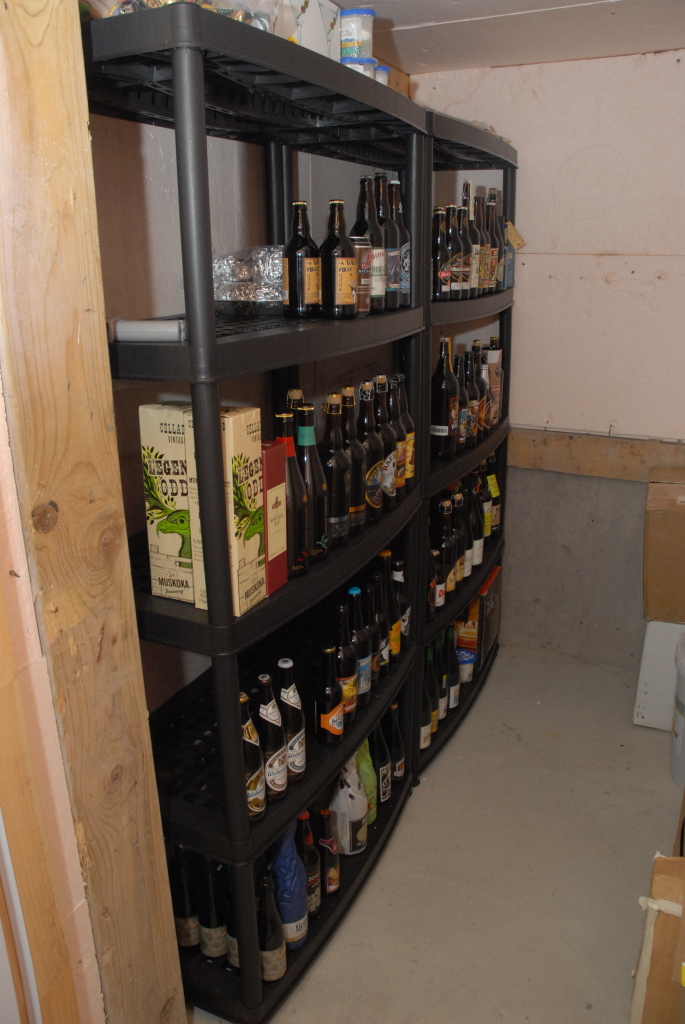This image, positioned horizontally, needs to be turned 90 degrees to the right to be viewed correctly. It is a poorly lit, full-color indoor photograph of what appears to be a small storeroom, perhaps a closet or pantry. The space has sheetrock walls descending to a concrete base and a low sheetrock ceiling. Featured prominently are two plastic shelving units with five rows each, filled with various bottled beverages that are likely alcohol. The bottles, which vary in size from approximately 10 to 16 ounces, are neatly aligned on the middle shelves, with some on the lower levels. Among the bottles are two distinct boxes: a white one with green and black printing, and a red one with a white label and additional text. The wooden door frame in the foreground accentuates the intimate, confined nature of the space.